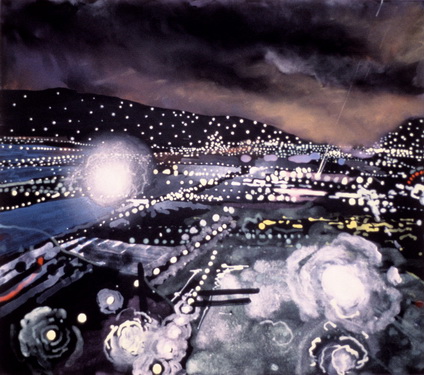The image is a detailed painting, likely done in acrylic, showing a nighttime urban landscape with a myriad of lights, creating a sense of bustling city life. The city lights are represented by numerous little circles, scattered in rows resembling streetlights and building lights. In the foreground, the buildings closest to us are depicted as unevenly sized white squares, while those farther away appear as basic blocks. Trees dot the scene, with some located at the bottom left and a large puffy white tree on the bottom right, depicted with a unique style reminiscent of tornado tops seen in weather reports.

The background features a black mountain ridge adorned with numerous lights, adding depth to the scene and blurring the line between natural and urban elements. The sky above is filled with dark, brooding clouds in shades of black, dark blue, and reddish brown, devoid of any lights, creating a stark contrast. Amidst the cityscape, two notable lights catch the eye: one on the left and another toward the bottom right, both surrounded by swirling white colors, suggestive of some form of electrical energy or sci-fi-like phenomenon. The foreground primarily showcases hues of blue, while darker tones dominate the background, enhancing the painting's dramatic and atmospheric quality.